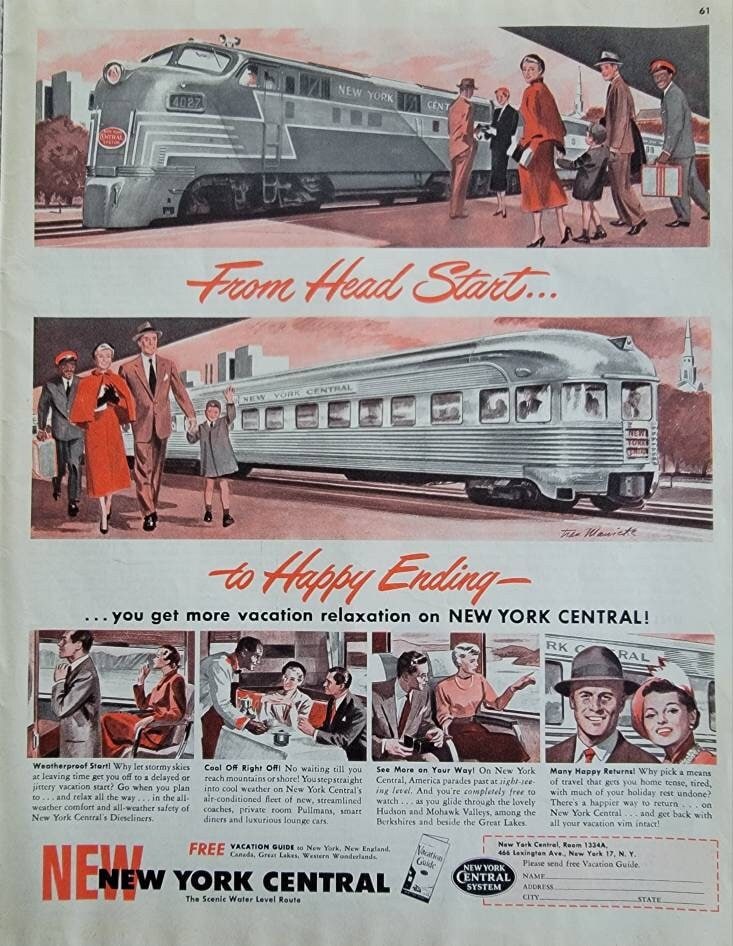The image depicts a vintage advertisement, possibly from an old newspaper or magazine, promoting the New York Central Railroad. In the top right corner, the number "61" is prominently displayed in black. The advertisement is marked by its aged, white, withered appearance and features a series of illustrated and drawn images.

The top section of the advertisement shows a silver train adorned with intricate detailing. Gathered around the train are people dressed in formal wear, including suits. Notably, there's a couple holding a child's hand and an old-school caricature of a Black person. Red text beneath this scene reads, "From Head Start." The next image portrays the same group of individuals walking past the train as it begins to move, with a young boy depicted waving. Below this, in red text, it reads, "To Happy Ending," followed by the phrase in black, “You get more vacation and relaxation on New York Central!”

The bottom section of the advertisement features four detailed illustrations of people enjoying different activities on the train: a man looking out the window, a couple being served, another couple gazing out the window, and a final couple posing for a photo. Small, hard-to-read text accompanies these images, offering further descriptions. Beneath these illustrations, bold text proclaims "New New York Central!", with the first "New" emphasized in red. To the right, there is a small form for readers to fill out their name, address, city, and state, suggesting they could receive additional information or a vacation guide.